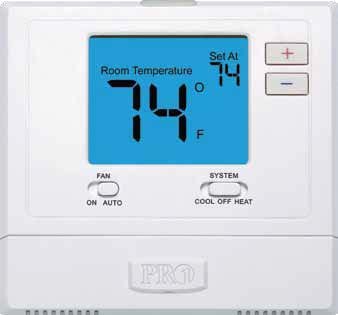This close-up image showcases a digital thermostat mounted against a pristine white background, creating an isolated focus on the device itself. The thermostat, a sleek eggshell white in color, prominently features a clear and easy-to-read digital display with a calming light blue, almost sky blue, hue. The display indicates the current room temperature is 74 degrees Fahrenheit and confirms that the system is set to maintain this temperature.

Located to the right of the temperature settings are two prominent buttons, marked with plus and minus symbols, likely for adjusting the desired temperature up or down. Beneath the central display, there are two essential slider switches. The left slider is set to 'Auto,' which manages the fan's operation but can also be switched to 'On' for continuous fan activity. The right slider, currently in the 'Off' position, governs the system's operational mode, allowing for toggling between 'Heat,' 'Off,' and 'Cool' settings.

The thermostat's brand, Pro, is subtly embossed in the same delicate eggshell white finish as the rest of the unit, adding a touch of elegance and ensuring brand visibility without disrupting the minimalist design.